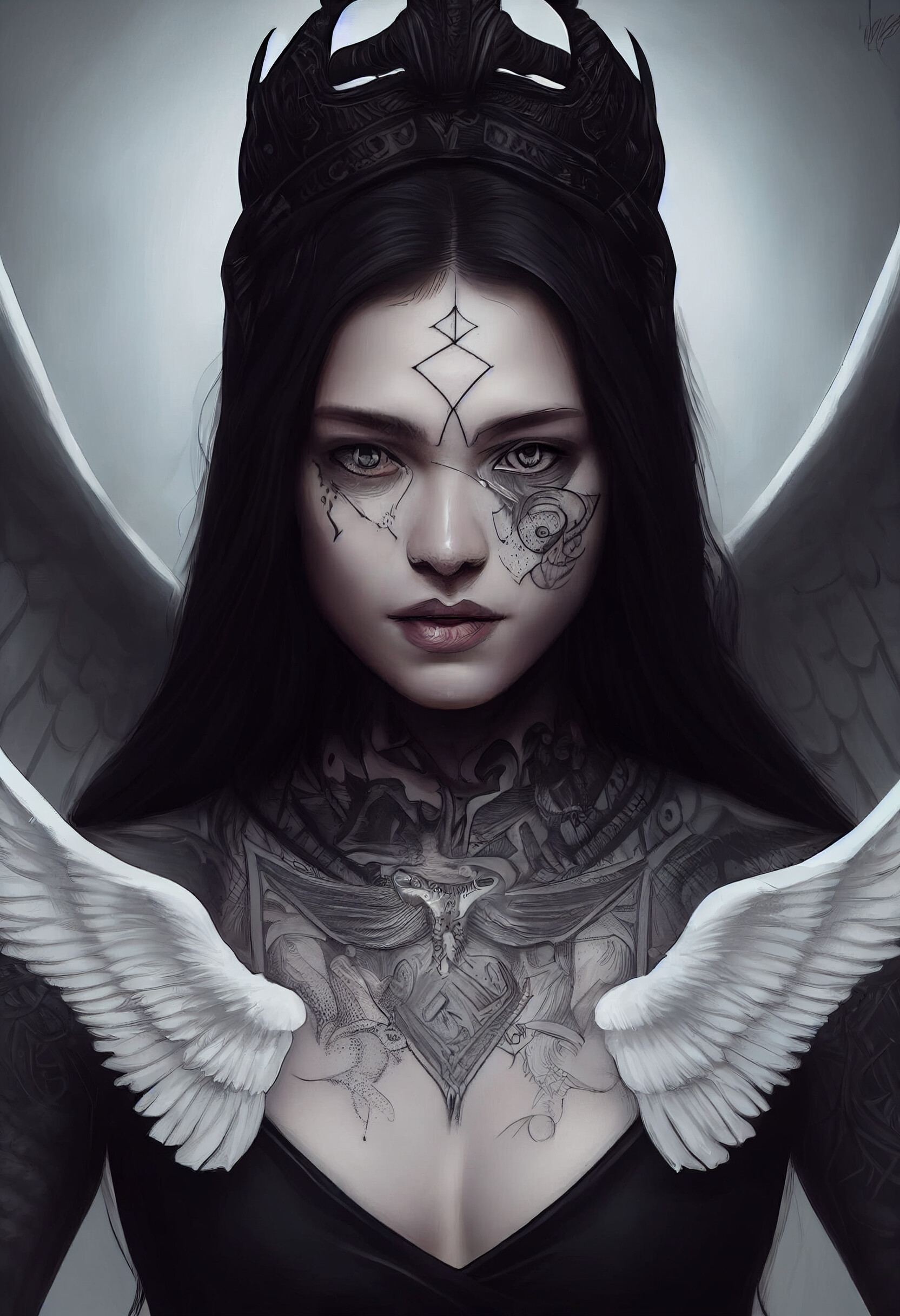This is a highly detailed digital image designed to resemble a realistic photograph, although it exhibits elements of illustrative artwork. The image depicts a woman with long, dark black hair neatly parted in the middle. She is adorned in a tightly fitting black V-neck tunic, which features a noticeable plunge down to the middle of her chest, exposing her neck and shoulders densely covered in intricate tattoos. 

Perched atop her head is a strikingly ominous black crown, adorned with pointed spikes and gray designs, giving it a menacing, demonic allure. Her face is distinctly pale, accentuating the black ink of her numerous tattoos. Vertical diamond-shaped tattoos embellish her forehead, with the top diamond split to point towards her hairline, and the bottom split to angle towards her eyebrows. Below her left eye, a cascade of tattoos extends in a necklace-like pattern, while her right cheek showcases a flower tattoo depicted solely with black ink lines.

Her eyes, which have been digitally altered to appear unnaturally clear, perhaps blue or green, add an otherworldly element to her visage. She wears light pink lipstick, enhancing her gothic aesthetic. Prominently featured tattoos extend from her neck up to her collar area, forming an abstract arrangement of angelic and demonic motifs.

Adding to her ethereal appearance, the woman has angel wings sprouting from her back, as well as smaller wings adorning each side of her chest at the collar. The backdrop further enhances the mystical aura, with a gradient halo effect transitioning from bright white behind her head to fading black, forming an almost divine illumination around her.